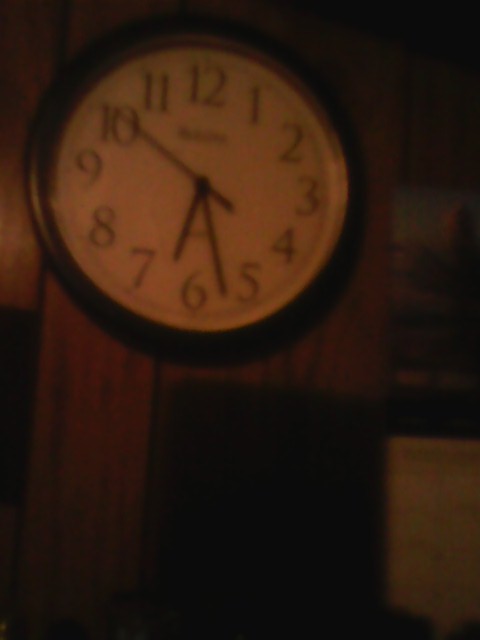The photograph, captured in low resolution and slightly taller than wide, depicts a wooden wall under mixed to dark lighting. The focal point of the image, occupying around 50% of the top left corner, is an analog clock. This white clock, outlined with a black trim, features prominent numbers 1 to 12 around its rim. The clock hands are clearly visible: the thin second hand points towards 10, the long minute hand is positioned between 5 and 6, and the short hour hand lies between 7 and 6, indicating a time close to 6:30. In the dimly lit background, a wall, possibly draped with a slightly yellowed curtain, is faintly discernible. The overall blurriness adds an enigmatic quality to the scene.